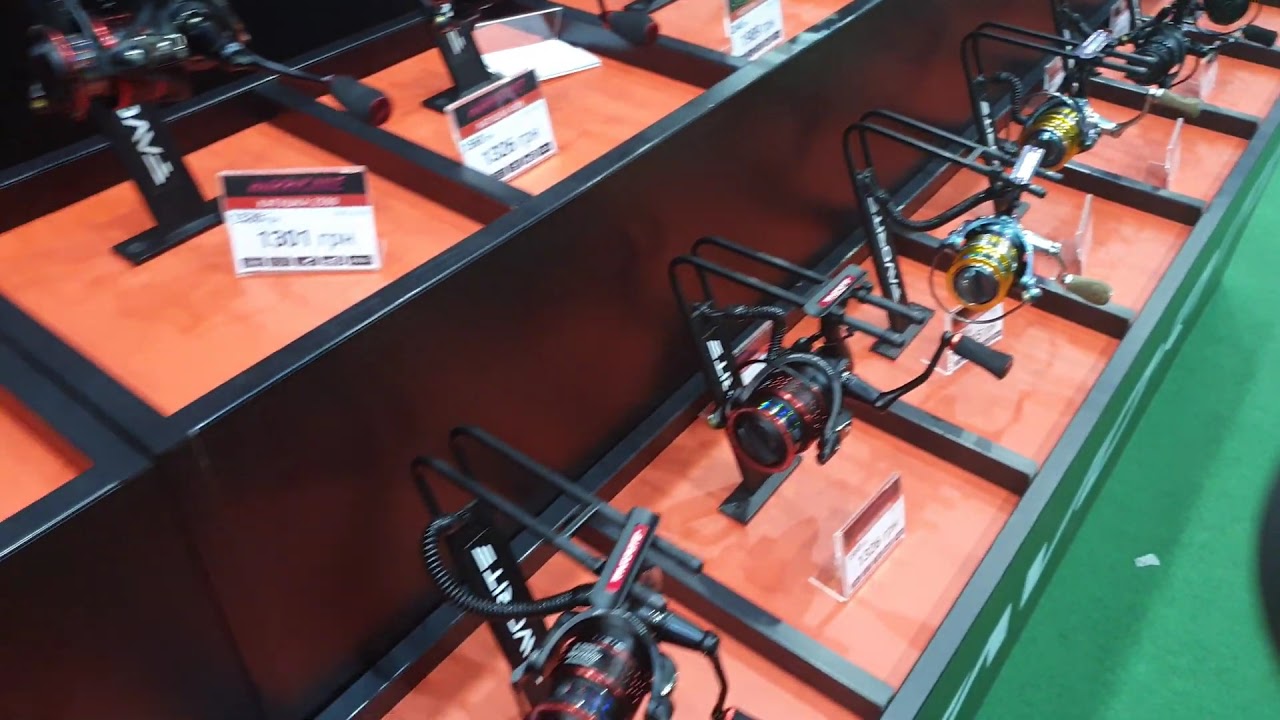The image portrays a sales event for camera equipment, captured from a top-down perspective. The primary focus is on two diagonal rows extending from the bottom edge to the upper right corner of the frame. Each row consists of items meticulously organized into small, black-framed rectangular sections with vibrant orange floors, each housing a camera or camera lens. Certain sections also feature placards detailing prices and sales information. The items, predominantly black, exhibit some variations with hints of red and yellow. Each camera or lens appears securely mounted on individual racks. Additional detailed elements include black, cylindrical items with red trimmings and wires, possibly indicating intricate camera components. A solid green area is visible on the right, contrasting with the organized array of camera gear.